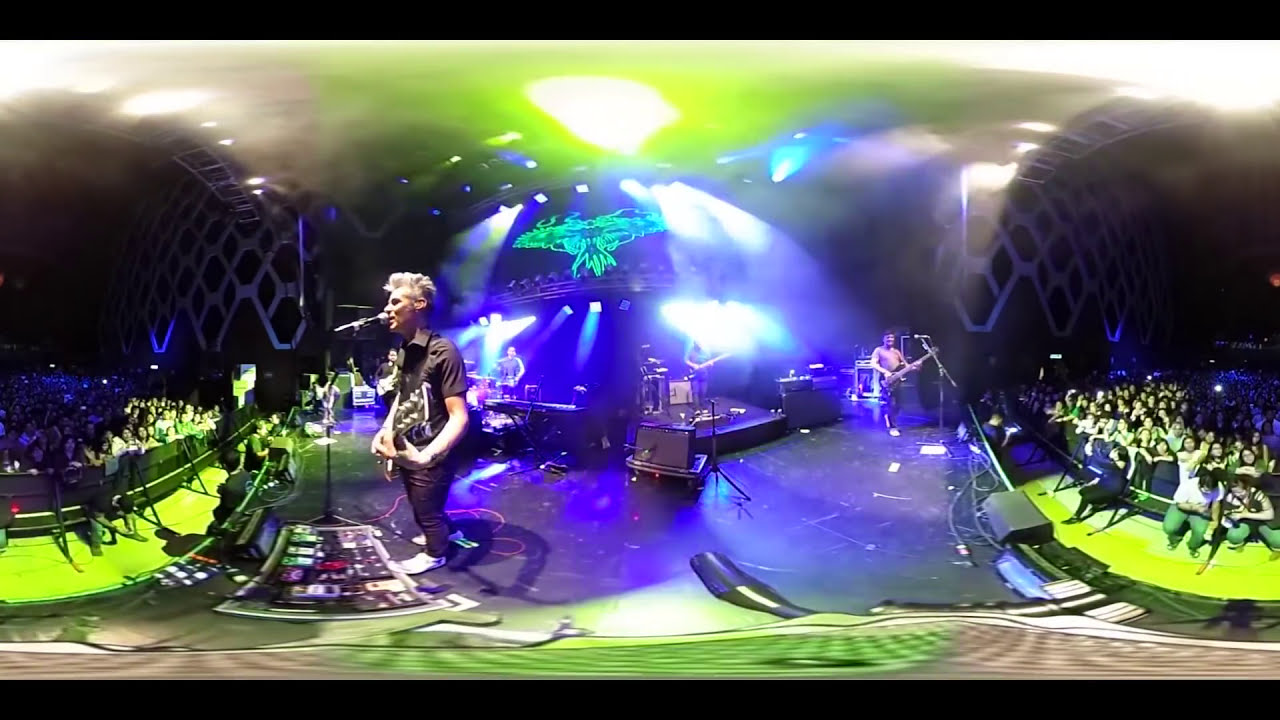This 360-degree panoramic image captures a live concert featuring an indie punk or alternative metal band. The stage is vividly lit with yellow and blue lights that reflect off a yellow ceiling and blue surrounding, creating a hazy atmosphere possibly enhanced by fog machines. Center stage, a graying yet spiky-haired lead vocalist, dressed in a short-sleeved button-up shirt and black trousers, sings passionately into a microphone while playing the guitar. Flanking the stage to the left, another musician, shirtless and in blue pants, energetically strums his black guitar. More towards the back, a drummer in a white shirt and dark pants keeps the rhythm steady. The stage is decorated with numerous devices featuring silver, red, purple, blue, and green buttons and stepping pedals. A striking characteristic of the image is the fisheye lens effect, evident from the curved mixing board in front and the seemingly distorted audience on either side. The crowd, bathed in a warm yellowish glow, appears engaged and enthusiastic. Despite the intricate detailing of a green symbol on a black background wall and white designs, the exact nature of the venue—whether indoor or amphitheater—remains ambiguous. Nonetheless, the packed audience suggests the band is well-known and beloved by many.